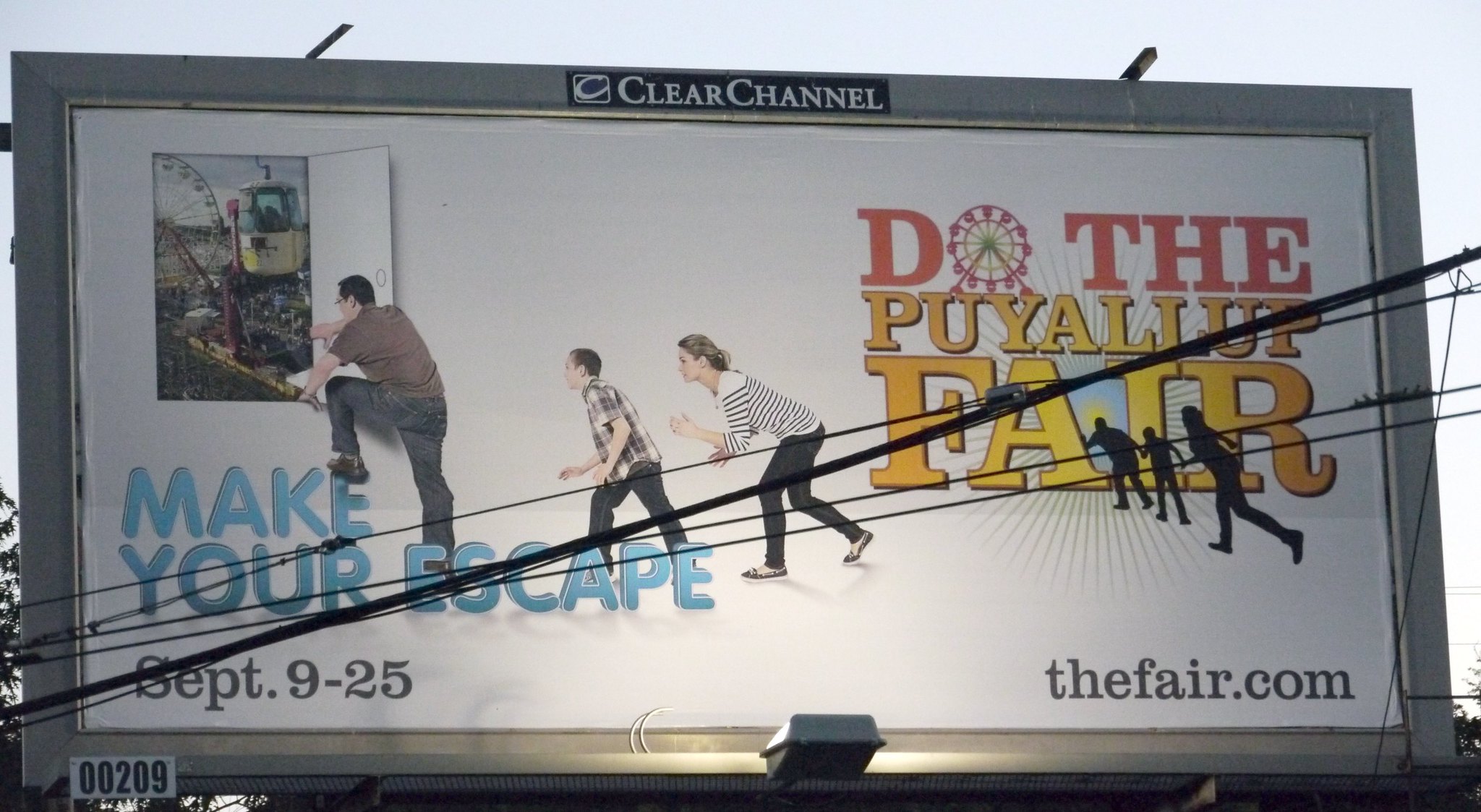This photo captures a large rectangular billboard set against a bright blue sky. The billboard features a dark gray border surrounding a white background. Dominating the lower left corner, in vibrant blue bubbly letters, the phrase "Make Your Escape" draws attention. Directly beneath this, the event dates "September 9th through 25th" are displayed in a bold black font.

Above the title and dates, the image depicts three individuals seemingly escaping from the stark white room depicted in the background. One man is portrayed climbing through what appears to be a window or door, emerging into a colorful carnival scene. 

On the right side of the billboard, in large lettering, it reads "Do the Puyallup Fair," emphasizing the name of the event. Positioned in the bottom right corner, the website "TheFair.com" provides additional information. Topping the entire scene, in the middle of the billboard's border, the text "Clear Channel" discreetly labels the advertiser.